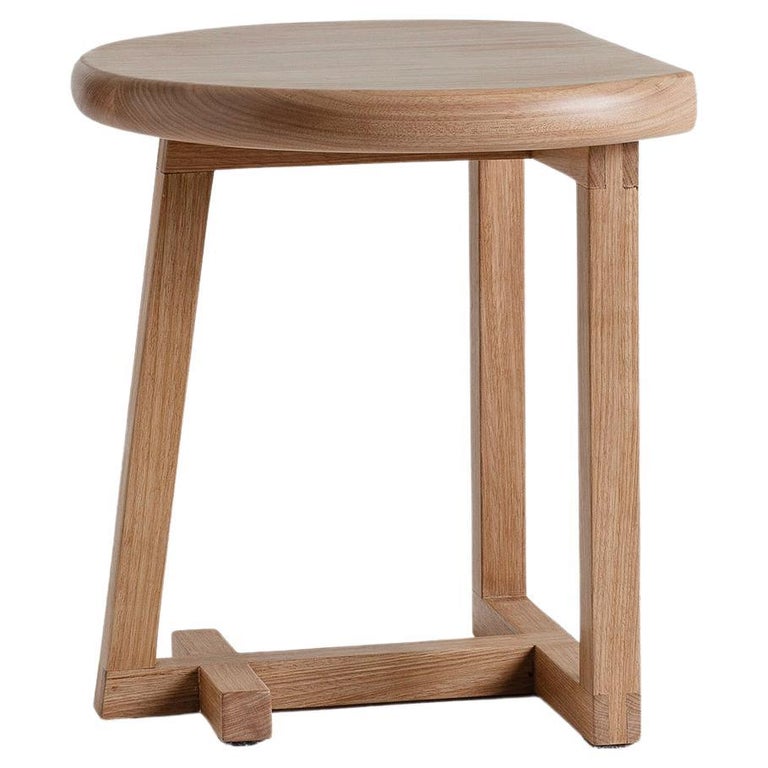This image features a wooden side table presented against a clean, white background, capturing every intricate detail. The table, made from honey-brown wood, reminiscent of oak, showcases a medium-tone finish that leans more towards the lighter spectrum. Its unique design includes a three-legged base, diverging from the conventional four-legged structure. These legs are interconnected by a cross-shaped support, adding both stability and visual interest. The tabletop itself is an unusual blend of shapes, with one side appearing circular, while the opposite side transitions into a squared-off edge. The high resolution and crispness of the image suggest a professional product photo, possibly intended for a catalog or an online store, emphasizing the table's design and craftsmanship.